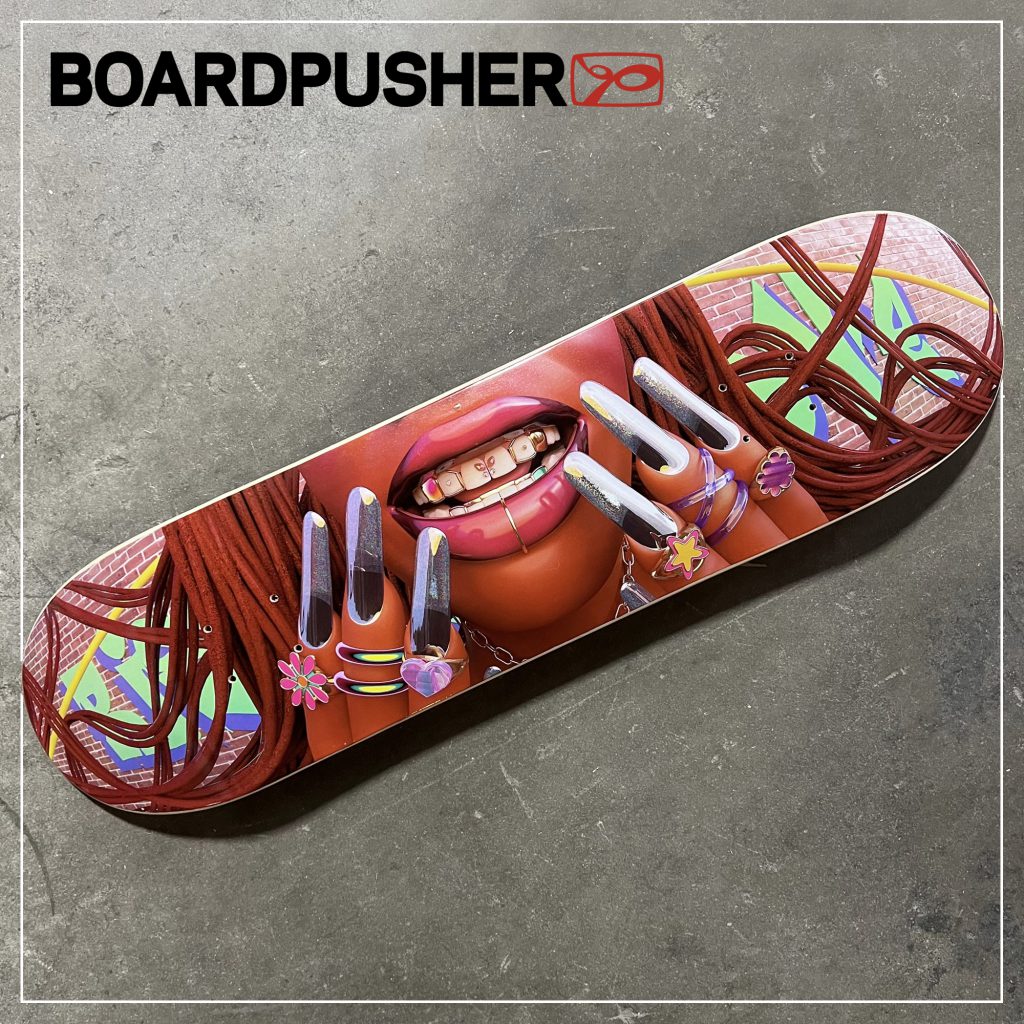The poster for "Board Pusher" prominently displays a skateboard deck set against a gray, weathered asphalt background with a thin square border. The deck is positioned diagonally and features a striking painting of a young black woman's mouth, adorned with gold and silver teeth and a lip ring. Her shiny, long metallic nails, decorated with rings, rise up to her face, with her fingers and nails in focus. Her lips are painted pink, contrasting with her intricate teeth artwork. Thin, brown braids frame the partially visible lower half of her face. At the top of the poster, "Board Pusher" is written in bold black letters, accompanied by a red, swirly logo. Behind the skateboard, a wall with graffiti adds to the urban aesthetic.